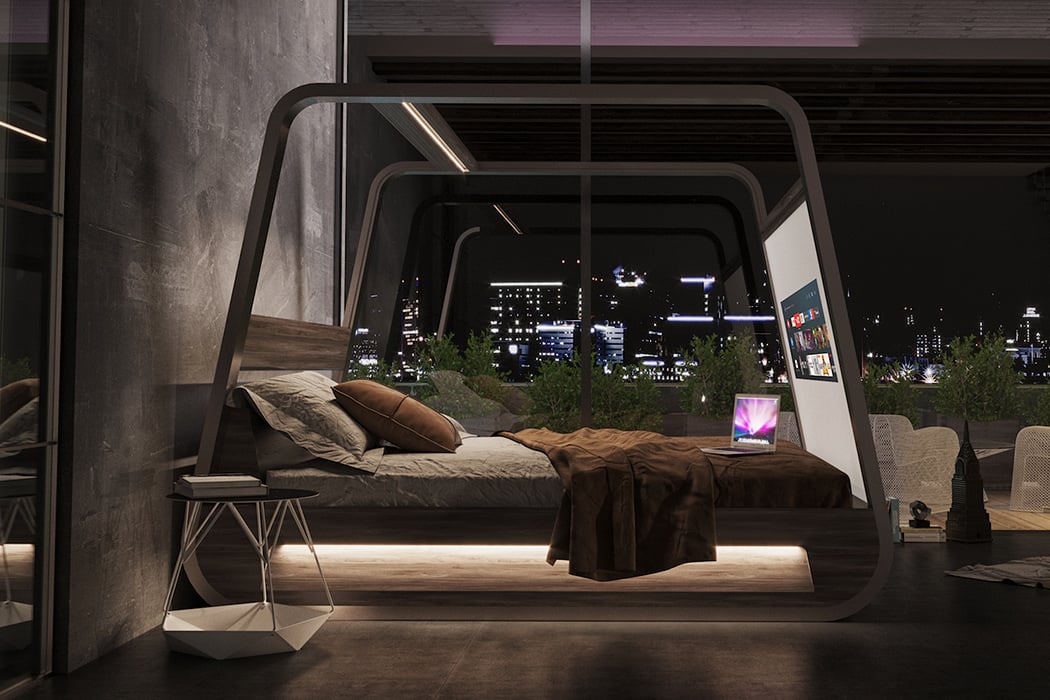This image showcases a highly futuristic and innovative bed situated in a modern bedroom. The bed resembles a canopy bed with a frame that extends from the headboard, arcs over the top, and culminates in a large screen at the foot of the bed. The headboard is a plain, horizontally oriented piece of dark brown wood, backed by a gray wall. The bedding includes brown pillows, brown blankets, and gray sheets, with a laptop resting on the covers.

The room features a simplistic nightstand next to the bed and is framed by large windows through which a cityscape is visible, illuminated by the lights of various buildings against a dark night sky. Green plants can also be seen outside, suggesting the presence of a terrace or balcony. The colors in the room are predominantly neutral tones—black, white, gray, and brown—with occasional accents of blue, green, red, and purple. The overall scene could either be an AI-generated rendering or a professionally taken photograph, emphasizing the novel concept of integrating modern technology into a traditional sleeping environment. The screen at the foot of the bed appears to function as an interactive display, possibly allowing access to various applications like YouTube, Hulu, and Peacock, turning the bed into a multimedia center. There are no people or animals present in the scene, and no discernible text is visible on the screen.